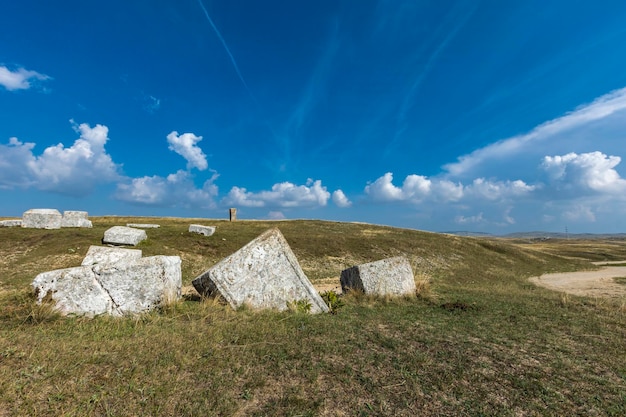In this photograph taken on a sunny day with a blue sky streaked by a few clouds, we see a large, grassy meadow dotted with historic ruins. Scattered across the field are six or seven large, weathered stone blocks, some cracked and slanted, and showing signs of age. The stones are predominantly grey but appear brighter under the sun's light. The meadow is mostly covered in short grass with occasional sandy patches, and on the right side, a dirt road or pathway is visible. In the distance, slightly left of center, a stone structure stands upright, resembling a tower. The scene is devoid of visitors, emphasizing the archaeological and historic nature of the site.